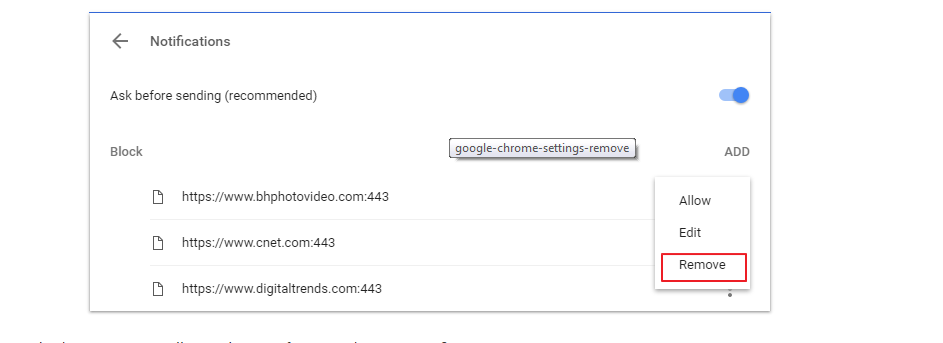This is a screenshot of the Google Chrome settings page, specifically focused on the Notifications section. The image is quite small, limiting the visible text. In the top left corner, there is a left-facing arrow (a back button), and next to it, the title "Notifications" is displayed. Beneath this header, there's an option labeled "Ask before sending (recommended)" with a blue toggle switch set to 'on,' indicating that the browser will request permission before sending notifications.

Below this setting, there's a column labeled "Block," which lists three URLs: "bhphotovideo.com," "cnet.com," and "digitaltrends.com." To the right of this column is an "Add" button. Between "Block" and "Add," there is a tooltip-like text, "google-chrome-settings-remove," appearing as if the cursor had hovered over an interface element, possibly due to a display glitch.

Additionally, a menu is open below the "Add" button, with options for "Allow," "Edit," and "Remove." The "Remove" option is highlighted with a red rectangle, indicating the user's current selection. The URLs listed under "Block" correspond to BH Photo Video, CNET, and Digital Trends.